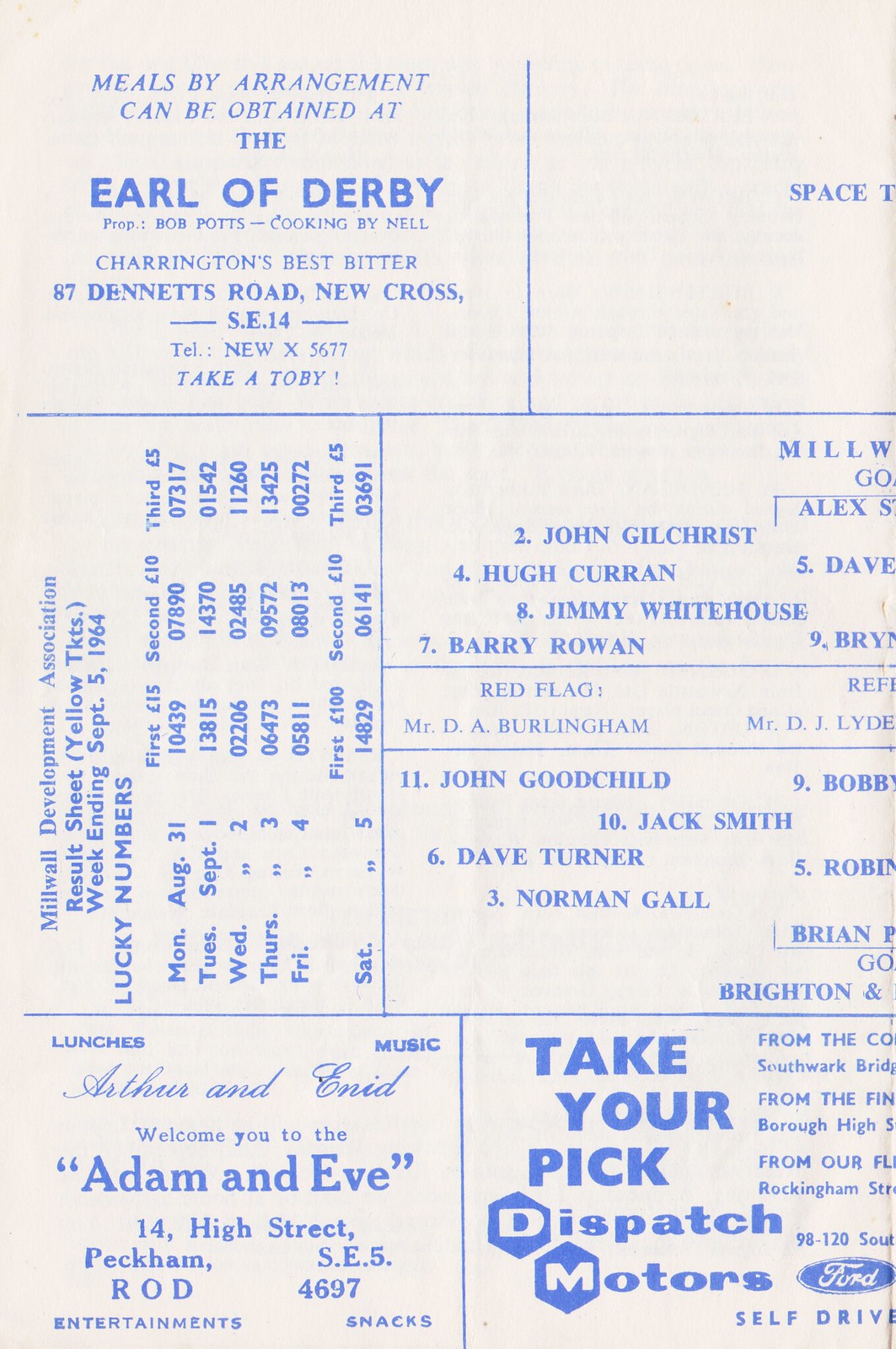The image is an old piece of paper, possibly from an old newspaper or poster, with a light grey or slightly pink background and text in blue ink. It comprises six columns, arranged in a 2x3 grid pattern with blue lines separating them. Each column contains rudimentary advertisements and textual information, indicative of a bygone era. 

The top left column features an ad that reads, "Meals by arrangement can be obtained at the Earl of Derby," followed by contact details: "prop Bob Potts, cooking by Nell, Charrington's Best Bitter 87, Denness Road, New Cross. SE14, tel: new X5677, take a Toby!" This suggests it is an advertisement for a restaurant. Other columns contain similar simple advertisements, one possibly for a rental car service, another for a play titled "Adam and Eve," and additional columns with names and statistics. There is also a table present in one of the middle columns, though the specific details within it aren't clear. The overall presentation is old-fashioned and text-heavy, indicative of historical advertising media.